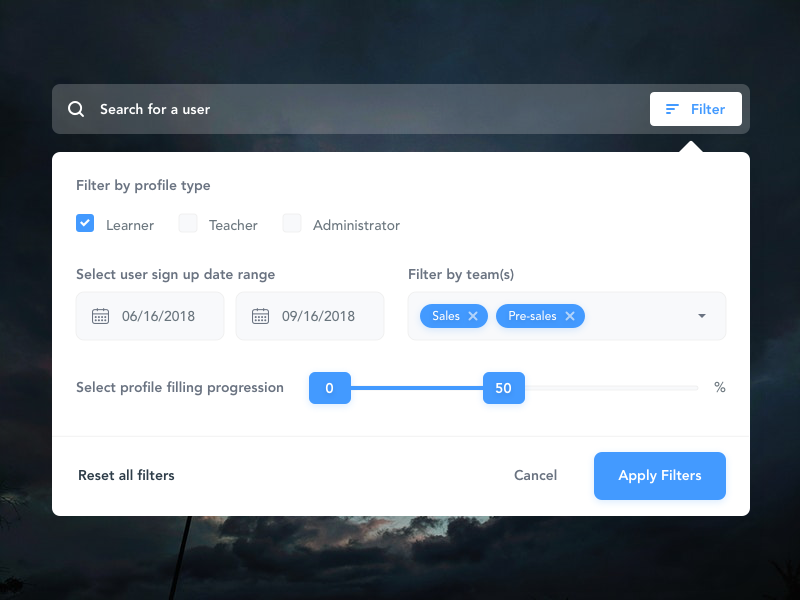The image shows a detailed interface of a filtering section. At the top, there is a search bar with the placeholder text "Search for user" on the left side and a "Filter" button on the right side. 

Below the search bar, the interface provides options to filter by profile type. There are three categories, each with a checkbox to its left: 

1. Learner (which is checked)
2. Teacher
3. Administrator

Further down, the interface allows the selection of a user sign-up date range, with the chosen dates being from June 16, 2018, to September 16, 2018. 

Next, it provides the option to filter by teams, with the available options being "Sales" and "Presales." 

There is also a "Select profile filling progression" feature, with a progression bar ranging from 0 to 50. 

Finally, there is a "Reset All Filters" option to clear all applied filters. This interface offers comprehensive and customizable filtering options for user management.